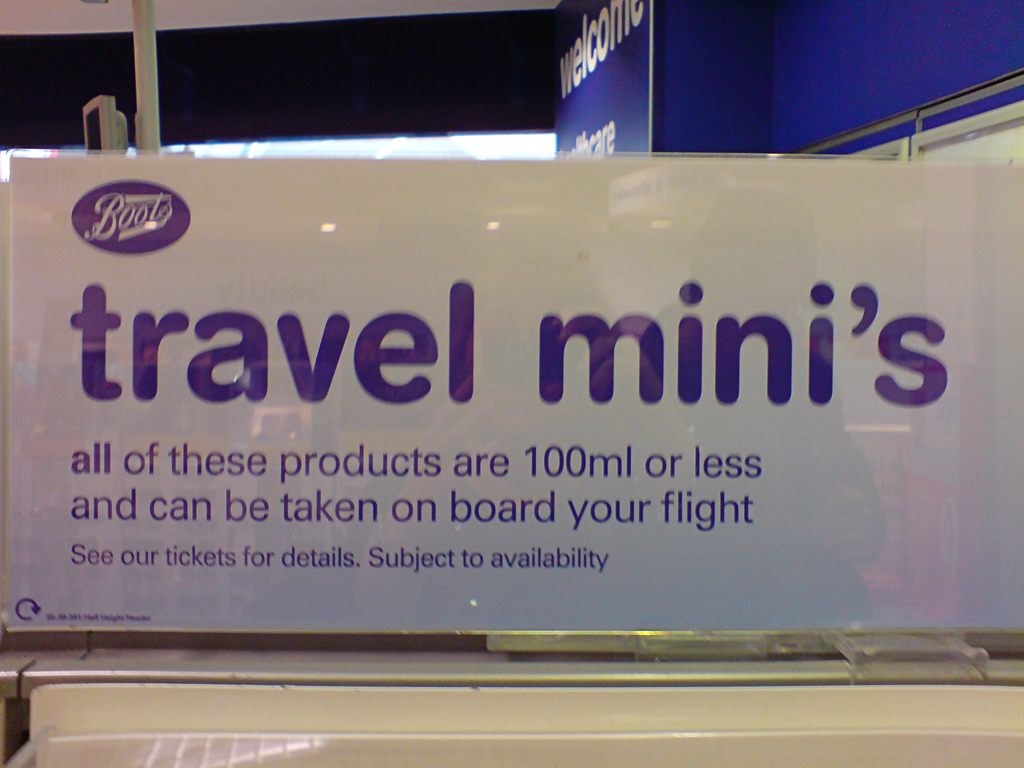The indoor photograph captures an advertisement sign encased in plastic. The sign prominently displays the phrase "Travel Minis" in large, purple lettering, followed by a note in smaller text: "All of these products are 100 milliliters or less and can be taken on board your flight. See our tickets for details. Subject to availability." Positioned at the top left of the sign is a logo reading "Boots" inside a purple oval. The sign's background is stark white with dark blue text, and its glossy surface reveals a faint reflection, suggesting the presence of the photographer.

Behind the sign, there's a vivid blue wall adorned with the word "Welcome" in white letters. Further to the center-left, partially obscured by the sign, is what appears to be a window. In the far top-left corner, just below the sign, a screen or monitor is visible. The sign itself seems to be placed on a metal table, indicative of an airport setting, enhancing the context of the travel-related advertisement.